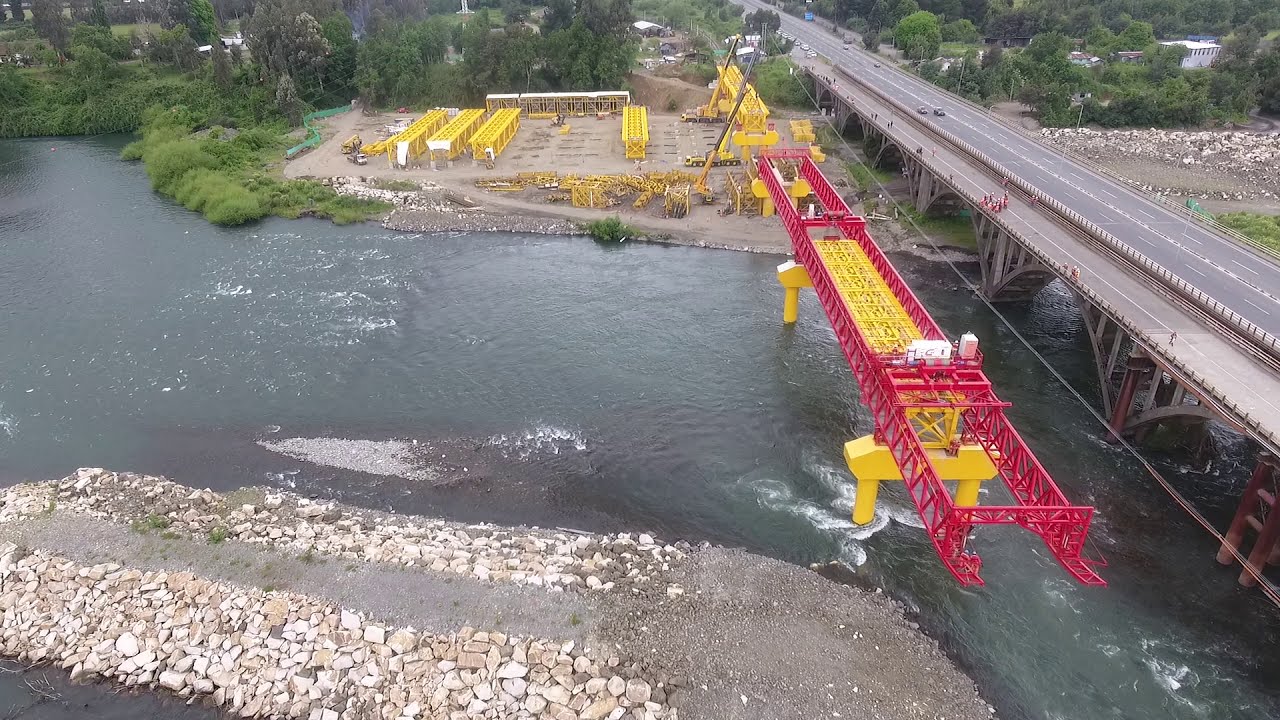This image captures an aerial, daytime view of a construction site by a river, highlighting a multi-lane overpass on the far right. This overpass, which has arched columns extending into the water and carries both vehicles and pedestrians, spans from the bottom-right to the mid-top of the photograph. Adjacent to the overpass on the left, there's ongoing construction featuring yellow and red metal scaffolding and boom work, indicative of a new bridge being built. The lower portion of the image shows a rocky embankment, while the cleared upper embankment on the opposite side of the river reveals additional yellow structural beams, suggesting further bridge construction. The background is lush with green trees, adding a natural frame to the industrial activity. The photograph is vivid with colors including yellow, red, green, gray, and blue, and despite the bustling activity, there is no text present within the image.